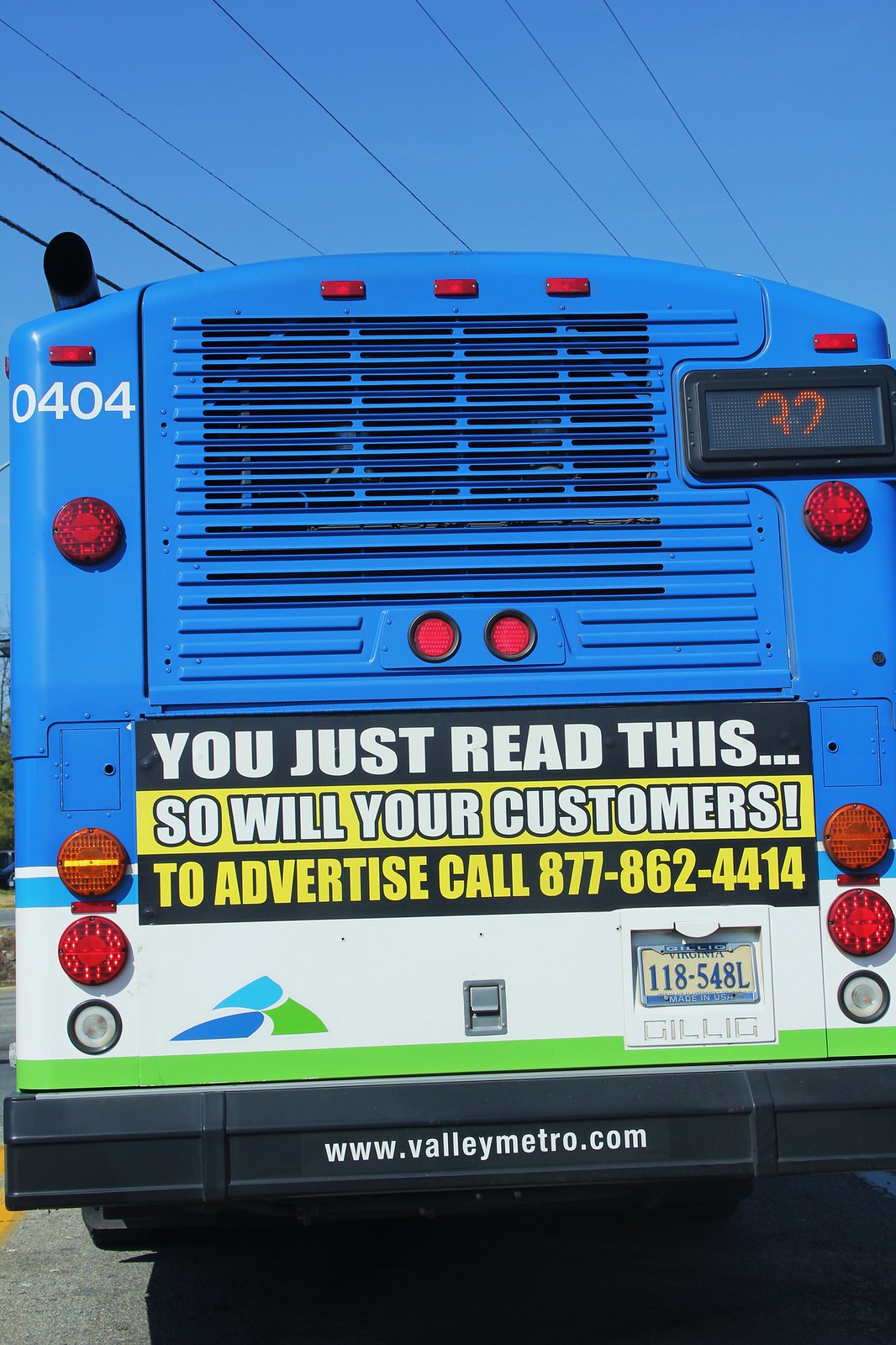This highly detailed photograph captures the back of a city bus bathed in sunlight under a clear, blue sky. The bus's upper half is predominantly blue, transitioning to white on the bottom half. Noteworthy details include the white number "0404" positioned in the top left corner. To the right of this number, a black LED screen displays the route number in vibrant orange, reading "32." A prominent banner adorns the lower half of the bus, characterized by black, yellow, and black stripes, bearing the text, "You just read this, so will your customers. To advertise, call 877-862-4401." The bus’s black bumper features the website "www.valleymetro.com" in white text. Also attached to the bus is a white Virginia license plate, numbered "118-548L." Reflective lights and markers are also visible, ensuring the bus is noticeable from behind.